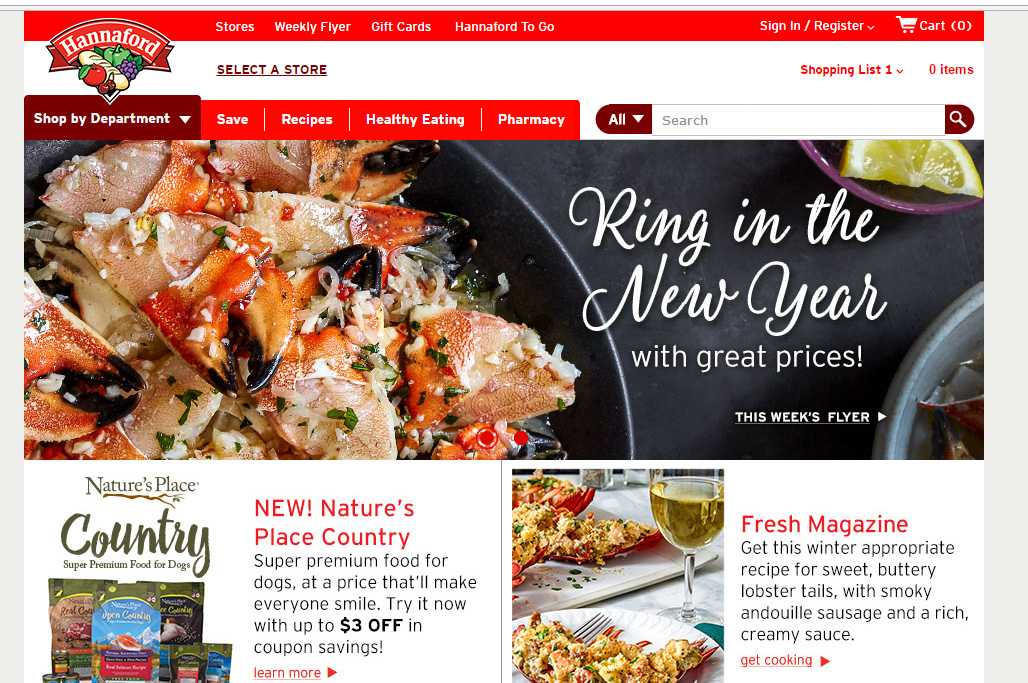**Website Homepage: Hannaford Grocery Store**

At the top of the webpage, a prominent red navigation bar provides quick access to key sections including "Stores," "Weekly Flyer," "Gift Cards," "Hannaford To Go," "Sign In," "Register," and "Cart." The Hannaford logo, consisting of a red banner adorned with the brand's name and illustrations of fruit and bread, is prominently displayed.

Beneath the logo, a link invites users to select their preferred store location. The main navigation menu offers options to "Shop by Department," "Save," "Recipes," "Healthy Eating," and "Pharmacy." A search bar is conveniently placed for easy product lookup.

An enticing image directly below these navigation elements showcases a delectable dish being cooked in a pan. The dish appears to be a flavorful mix of seafood, rice, vegetables, and various seasonings. Accompanying text reads, "Ring in the New Year with Great Prices." The image also features a dish garnished with lemon slices.

To the left of this enticing visual, an advertisement promotes "Nature's Place Country" – a new line of super-premium dog food. The ad highlights savings of up to $3 with coupon discounts and encourages users to try it now.

Adjacent to this is a promotion for "Fresh Magazine," inviting users to discover winter-appropriate recipes, such as sweet buttery lobster tails, perfect for indulging during the colder months.